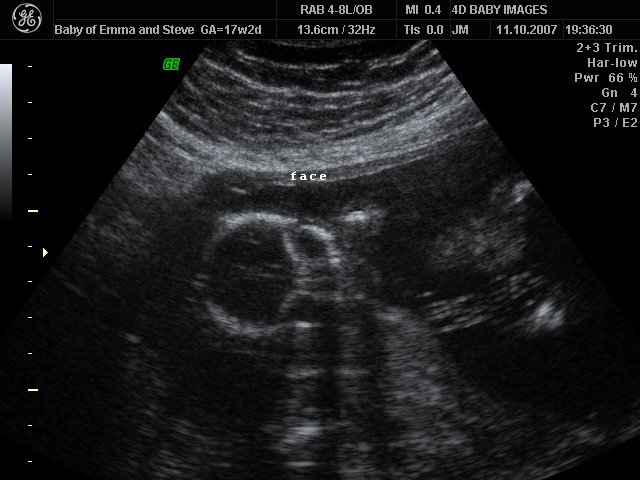This image shows a sonogram of a baby with a predominantly black and white color scheme, characteristic of ultrasound imagery. In the upper left-hand corner, there's a General Electric logo, indicating the manufacturer of the ultrasound machine. To the right of the logo is the text: "baby of Emma and Steve, GA=17W2D," which signifies that the gestational age is 17 weeks and 2 days. 

Further to the right, the top of the screen features the text "RAB4-8L/OB" and below this, "13.6 centimeters/32HZ." On the left-hand side of the image, more details such as "MI 0.44D baby images" and various strings of numbers and letters appear, including "TIS 0.0," "JM 11.10," and "0.207 19:36:30." Additional text includes "2+3 trim," "Harlow," "power 66%," "GN4," "C7/M7," and "P3/E2."

The ultrasound image itself is dark with a somewhat blurry and nebulous quality, typical of sonograms. In the center, white text labels a part of the image as "face," where a vague round shape can be discerned, suggestive of the baby's face with possible indications of the eyes, nose, and mouth. Other indistinct shapes around this suggest the baby's body, with a floating structure that is likely the placenta visible underneath.